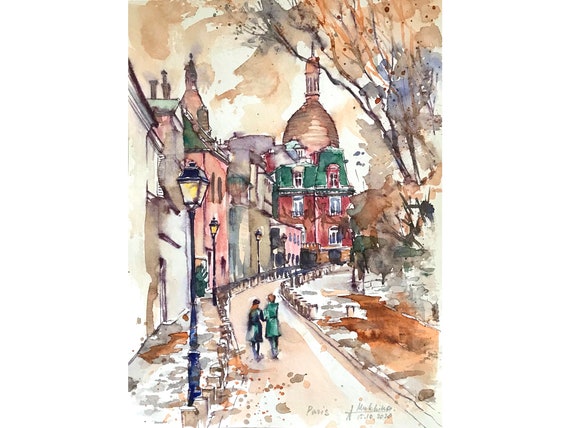This piece of watercolor art showcases a picturesque scene seemingly set in a quaint European town. The colors are bright yet somewhat muted in the foreground, transitioning to more vibrant reds and greens towards the background. The focal point of the painting is a couple walking down a sidewalk lined with slightly weathered buildings in hues of pink, red, green, and beige. 

In the center of the scene, one person, slightly taller and wearing a green coat, walks alongside a female companion dressed in a dark, long black coat. The setting suggests a chilly autumn or winter day, with a light dusting of snow on the ground. To the right, several trees add an element of natural beauty to the urban landscape, while a steeple rises in the distance, enhancing the idyllic charm of the town.